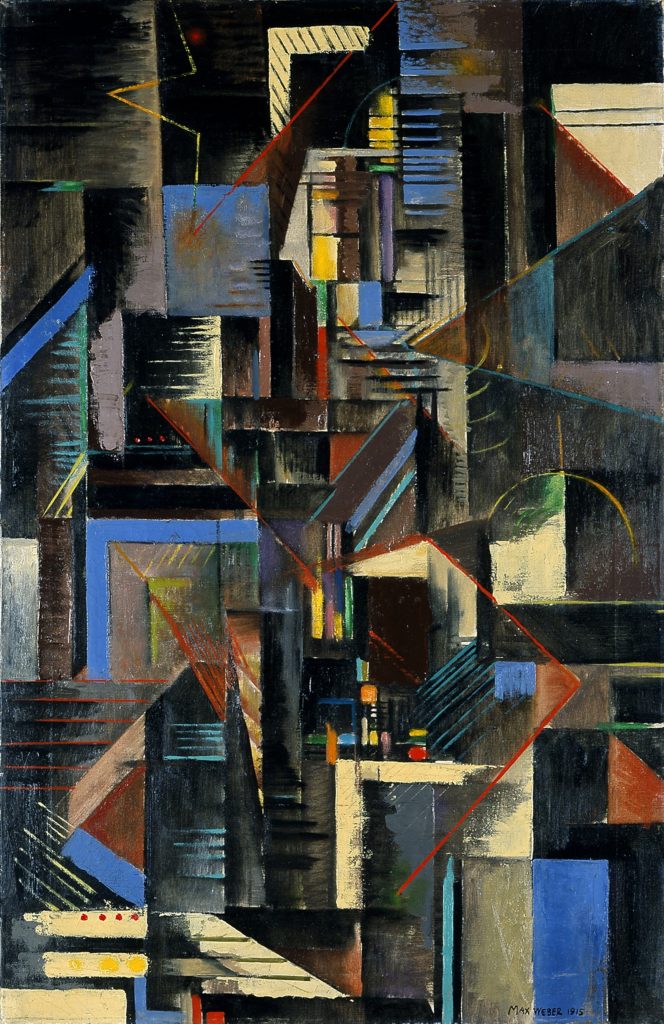This is an abstract oil painting by Max Weber, dated either 1912 or 1950, signed in black ink in the bottom right-hand corner. It features a vibrant and diverse palette, with predominant colors including various shades of blue, gray, white, red, yellow, green, and black. The composition is a dynamic interplay of geometric shapes—triangles, squares, and rectangles, with lines intersecting at various angles.

In the upper left corner, a black square transitions into a lighter gray with a striking yellow V-shaped line cutting through it. Adjacent to this area is a red line that intersects an angled yellow section filled with black lines, leading down into a blue square with a brown blotch and red lines. The painting also includes numerous patches of black, yellow, green lines, and colored bars scattered throughout.

At the bottom left, tiny yellow rectangles host distinct red and yellow dots—one with four red dots and another with three larger yellow dots. This detailed use of contrasting colors and dynamic shapes embodies the essence of abstract art, creating an engaging and visually stimulating composition.